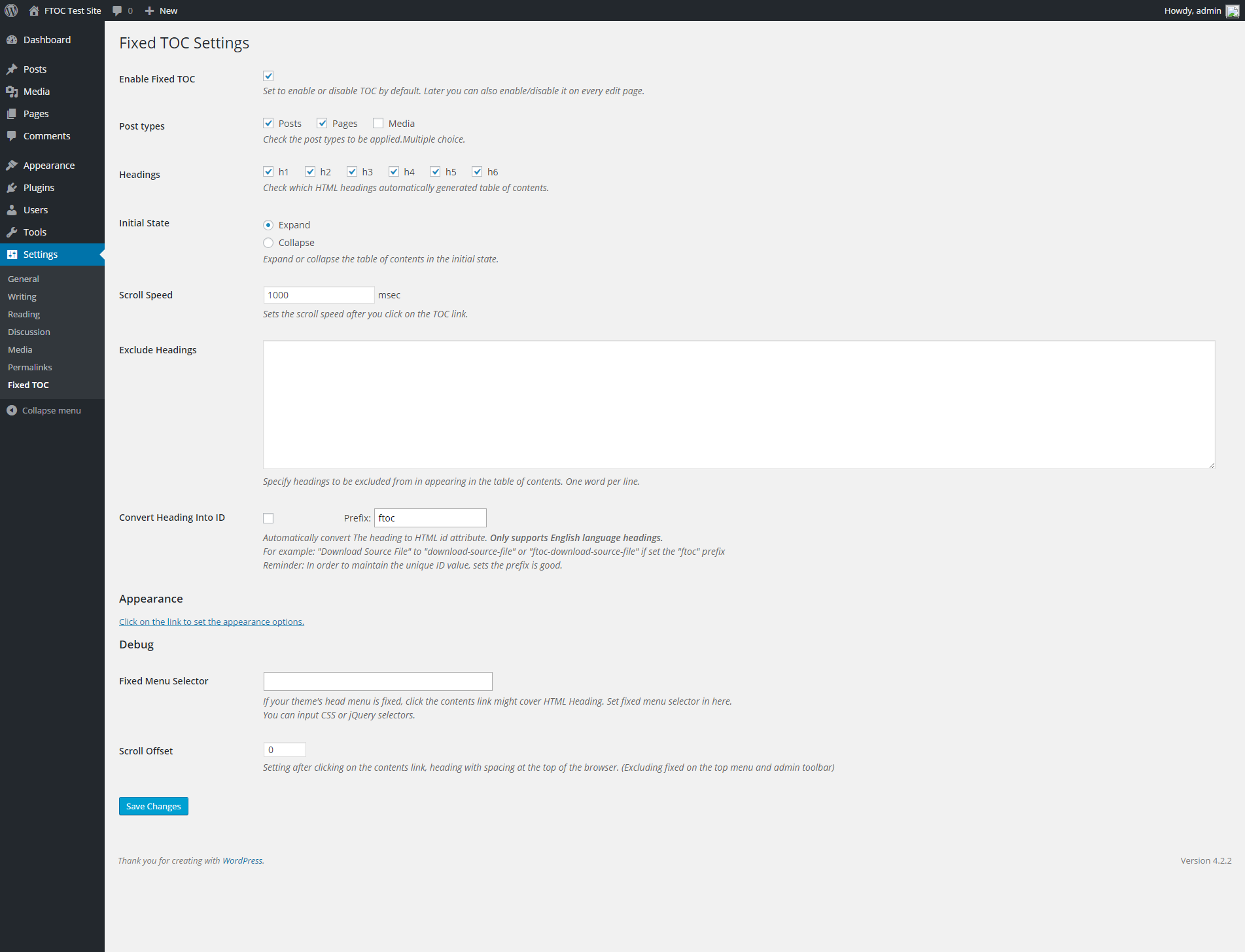This image depicts the detailed layout of an admin dashboard on the FTOC test site. At the top left corner, there's a logo followed by the home button. Adjacent to it is a "W" emblem, and to the far right, there is a "Howdy, admin" greeting indicating that an administrator is logged in.

Below the header, on the left-hand side, a vertical black column lists various menu items such as Dashboard, Posts (with a pen icon), Media, Pages, Comments, Appearance, Plugins, Users, Tools, and Settings. The 'Settings' section is expanded, revealing sub-options like General, Writing, Reading, and Discussion. The currently active section, highlighted in blue, is 'TOC Settings'.

The main content area on the right is focused on the 'Fixed TOC Settings'. A checkbox indicates that the 'Fixed TOC' feature is enabled. The settings are categorized as follows:

- Post Types: Options available are Posts, Pages, and Media, with Posts and Pages currently selected.
- Headings: All heading tags from H1 to H6 are checkmarked.
- Initial State: Set to 'Expand', with the alternative option to collapse.
- Scroll Speed: Set to 1000 milliseconds.
- Exclude Headings: The corresponding input box is empty.
- Convert Heading: This option is checkmarked.
- Appearance: A hyperlink directs to further customization options.
- Debug: Includes 'Fixed Menu Selector' (currently blank) and 'Scroll Offset' (set to zero).

A prominent blue "Save Changes" button is placed at the bottom for applying configurations.